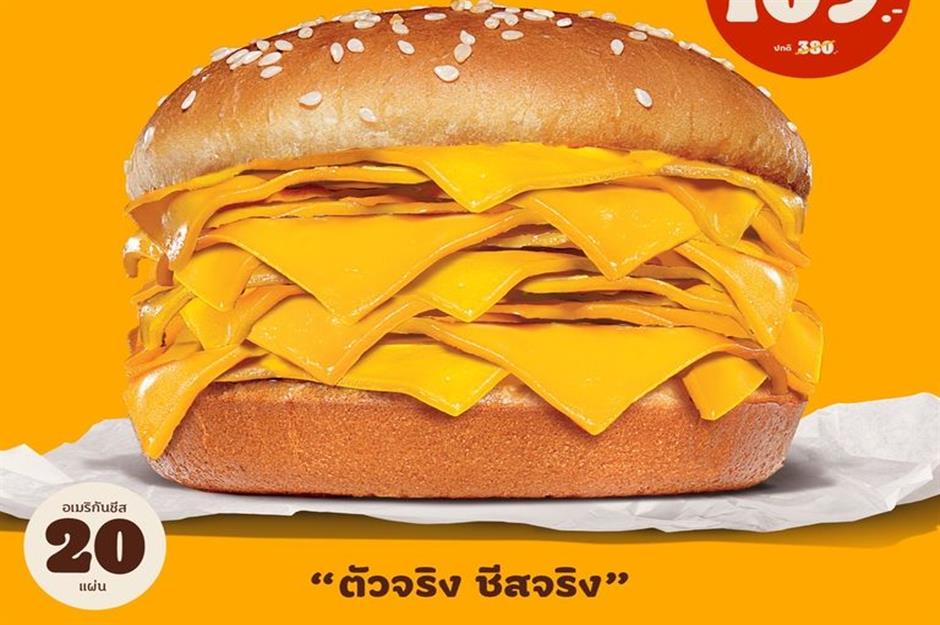The image depicts a visually striking sandwich that harkens back to the style of vintage Burger King advertisements. This unlikely creation consists of two sesame seed buns encasing an impressive stack of approximately 12 slices of square Kraft American cheese. The sandwich rests on a white wrapper, and the background is a matching cheese-colored hue, emphasizing the overwhelming presence of cheese. In the bottom left corner, a red advertisement price of "20" can be seen within a circle, accompanied by unrecognizable text in a foreign language, hinting at a surreal, perhaps AI-generated, context. The inscrutability of the language adds to the overall curiosity of the image, which prominently features cheese in lieu of any meat, making it a visually memorable yet perplexing take on a burger.